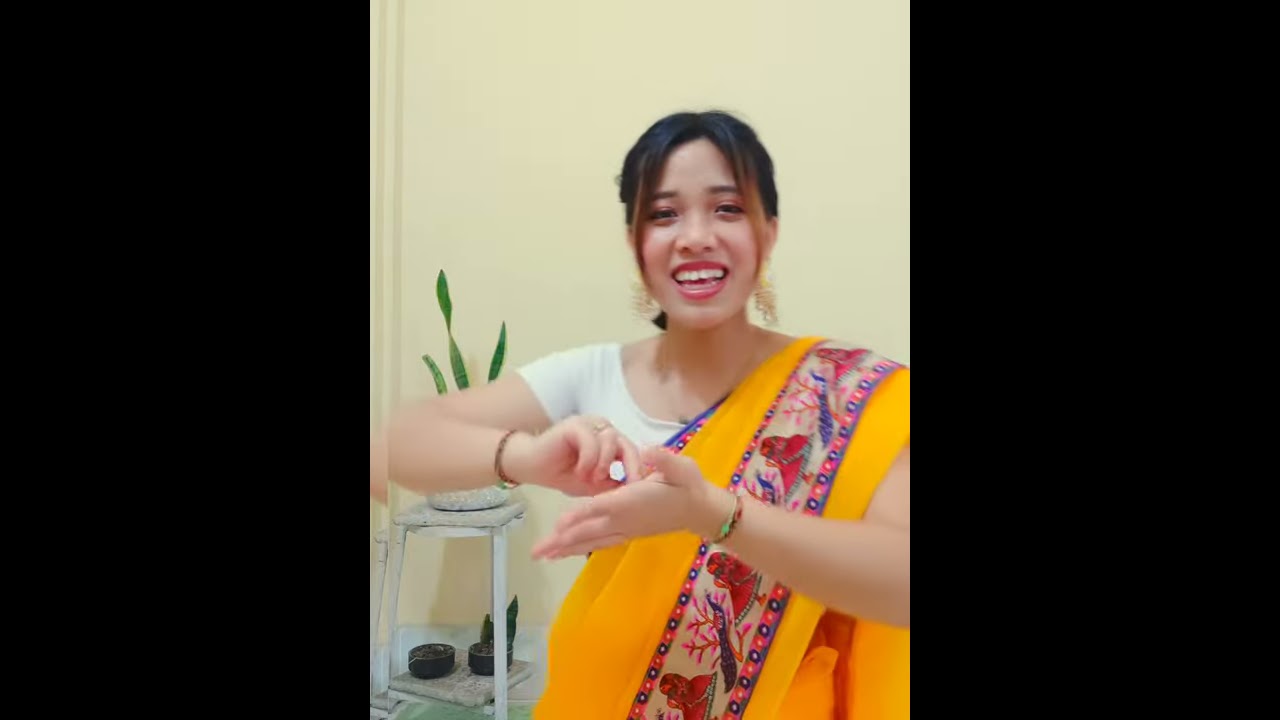The image captures a young Asian woman, likely in her 20s, with a joyful expression and vibrant smile, showing her upper and lower teeth. She stands facing forward with her hands raised in a gesturing motion, resembling a sign language gesture. She has dark, nearly black hair with light brown-blonde and orange tips on the strands framing her face, while the rest is pulled back. She is adorned in a white short-sleeved t-shirt over which she wears a bright yellow sari-like sash decorated with intricate red and blue patterns, including designs of a peacock and a woman in red. Her accessories include noticeable dangly golden earrings and bracelets on both wrists. The background features a beige wall, a white end table with a green potted plant, and additional potted plants underneath, all framed by thick black borders on either side of the image.